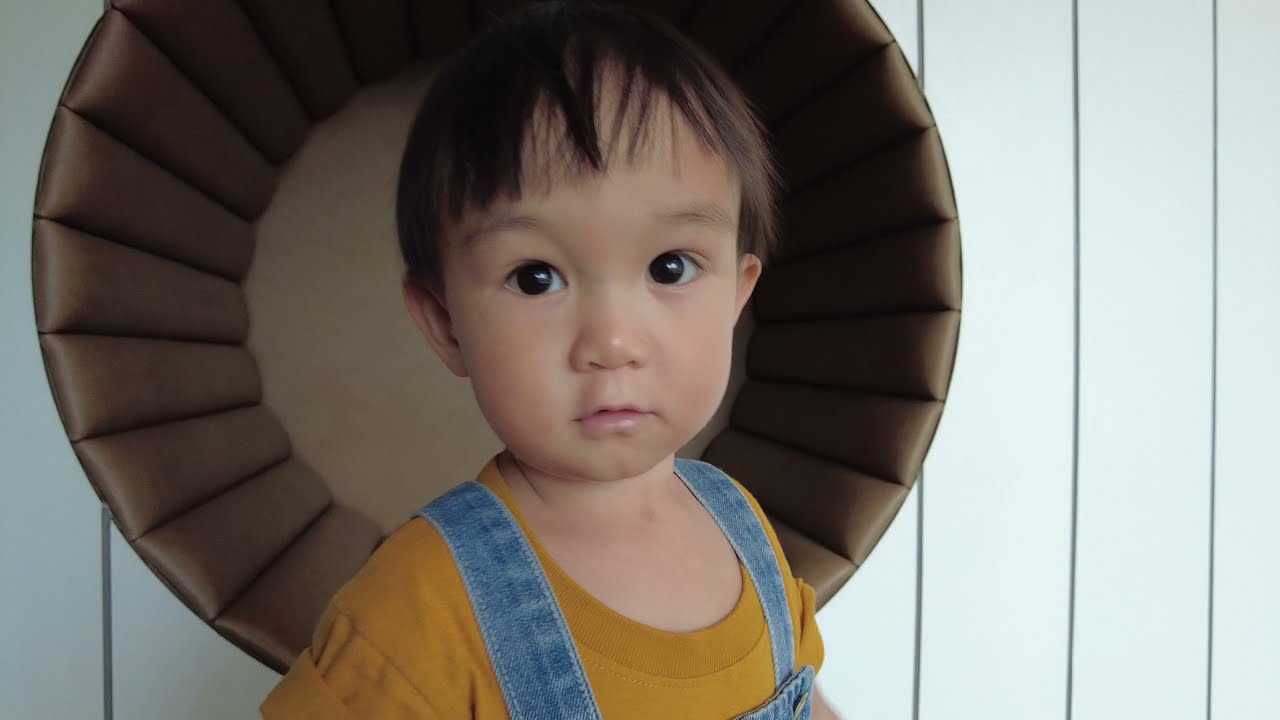The photograph features a young Asian child, approximately two years old, standing against a white, vertically-paneled wall. The child's dark brown hair is cut short, at the length of his eyebrows, giving him a straightforward and tidy appearance. He has large, dark brown eyes, thin eyebrows, a small button nose, thin lips, and rounded cheeks, with his mouth slightly parted. He is clad in a mustard-colored shirt underneath denim overalls that showcase a gold or silverish button at the straps. Behind him is a noticeable circular object, brown in color and possibly fashioned from paneled wood, resembling a cat cubby or an ottoman turned into a wall-mounted seat or perch. The child stands front-facing, expression neutral, neither smiling nor crying. The image captures him from the chest upwards, emphasizing his contemplative gaze directed at the camera.